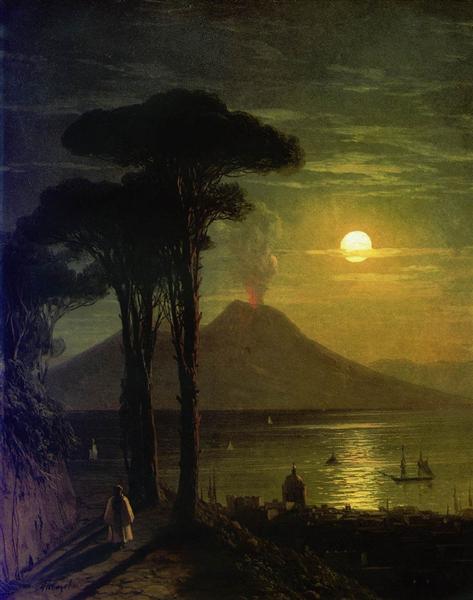The painting vividly captures a major volcanic eruption dominating the center of a vertically aligned, portrait-style oil canvas. The eruption itself is significant but not overly violent, with smoke and fire billowing from the volcano's peak. In the background, the sun, obscured by volcanic gases, hovers just above the horizon, giving the scene an eerie, dim glow that almost mimics nighttime. 

In the mid-ground, large, dark trees frame the scene on the shoreline, where a small, robed figure stands, gazing at the volcanic spectacle. This figure, along with the elevated viewpoint, suggests a vantage point approximately 50 feet from the immediate foreground. Below, a small city or town lies shrouded in darkness, nestled by the water's edge. 

On the lake between the town and the volcano, several details can be observed: buoy-like objects float on the water's surface and at least one canoe is visible, manned by two individuals. The color palette of the painting is rich and varied, transitioning from the yellow of the sun and the red of the volcanic fire to the brown of the ground and the grayish tones of the volcano, with a curious greenish tint infusing the sky around the sun. This nuanced interplay of colors and elements heightens the dramatic impact of the scene, encapsulating both the beauty and the destructive power of nature.